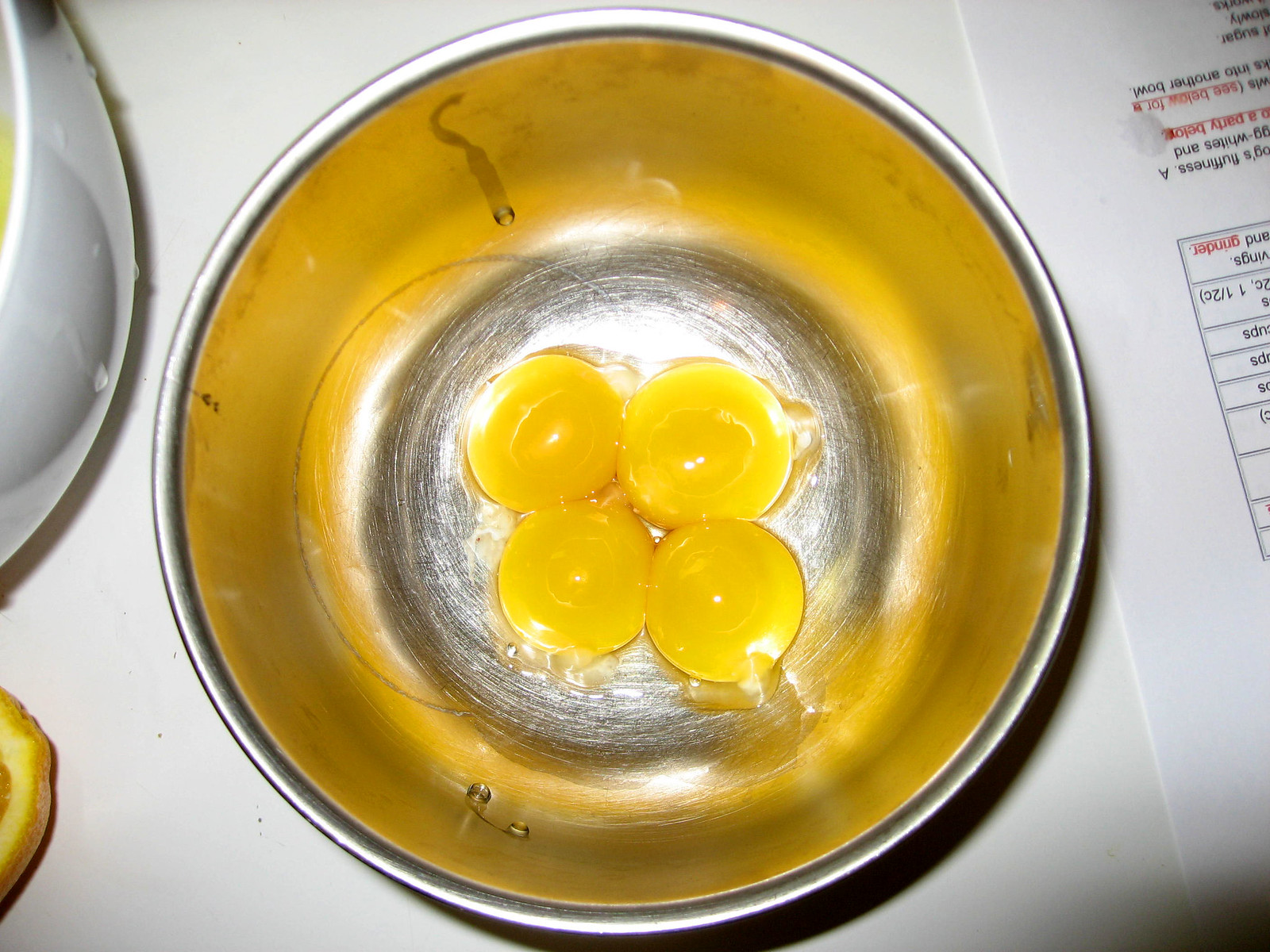This photograph, taken from directly above, showcases four intact, yellow egg yolks in a deep silver mixing bowl, reflecting the overhead light. The bowl is resting on a white countertop. At the top left of the image, part of a curved, white ceramic bowl is visible, though its contents are not. Just below, the textured rind of a halved orange can be seen in the bottom left corner. The right edge of the photo features a printout of a recipe, arranged with small boxes of text and hints of red and black ink, though the text is upside down and unreadable.